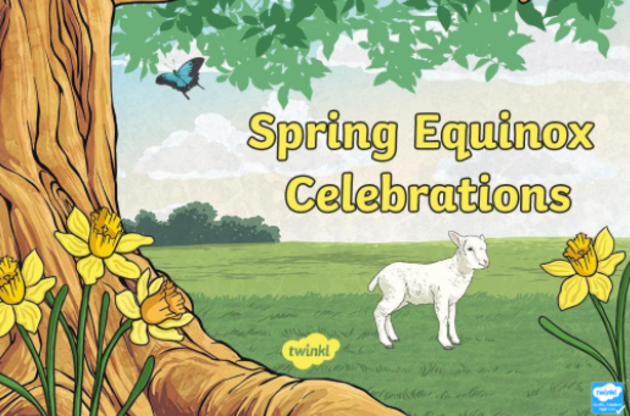This detailed illustration depicts a vibrant scene celebrating the spring equinox. Central to the image is a small, white lamb standing in profile on a grassy field. On the left side, an up-close view of a tree trunk with roots stretching into the grass is visible. At the base of the tree, three vibrant yellow daffodils with deeper yellow center cups and lush green leaves stand out. A solitary daffodil mirrors these on the bottom right of the image. Above the scene, green leaves hang down with a blue butterfly with black edged wings fluttering near the tree. The entire illustration is topped with the title "Spring Equinox Celebrations" printed in bold yellow letters outlined in black. Additionally, the logo "Twinkl" appears just below the lamb on the left and again at the bottom right in a blue and white design. The backdrop features a silhouette of distant trees, enhancing the sense of an open, lively field basking in the renewal of spring.